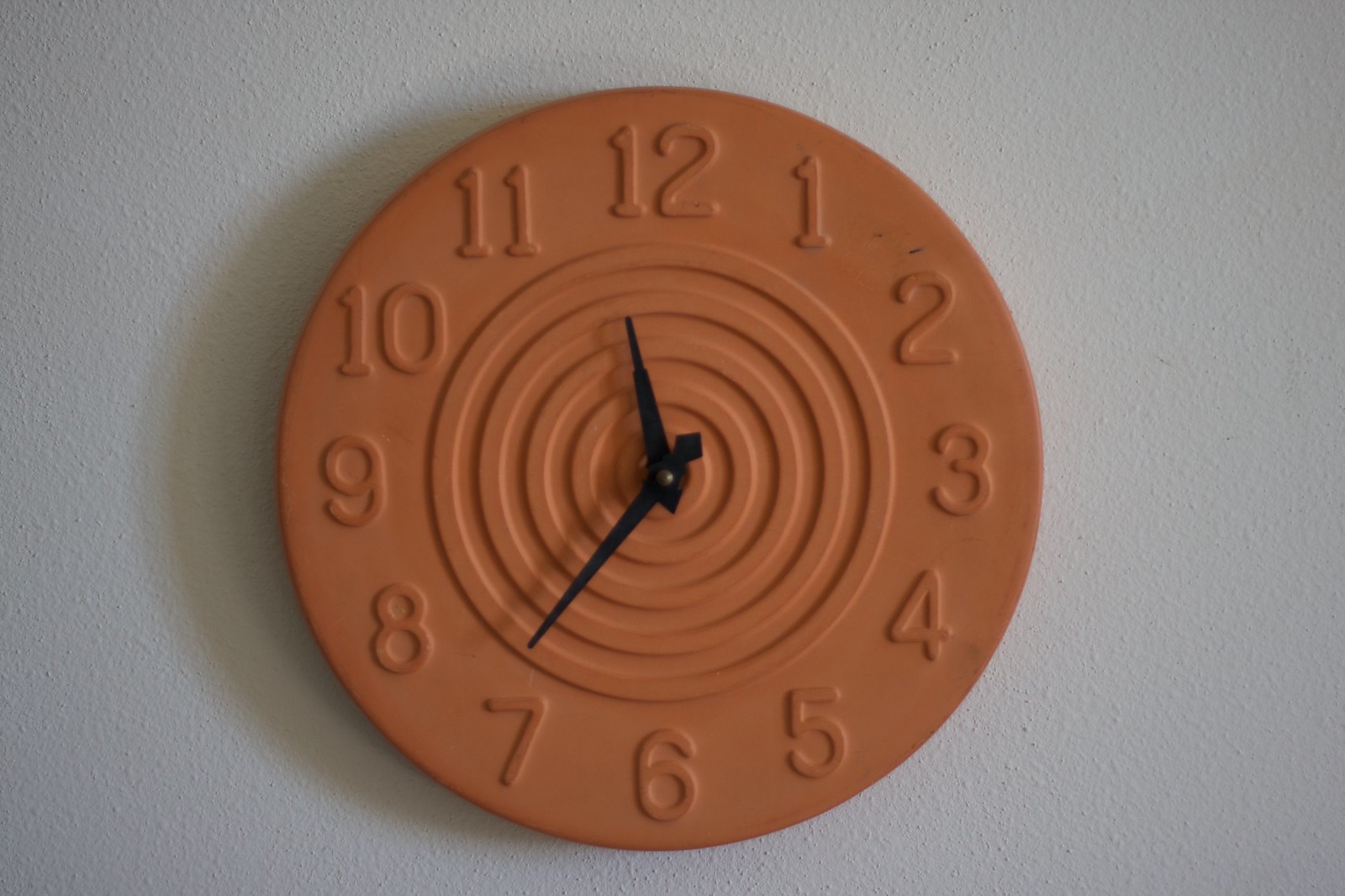This image depicts a terracotta clock showing the time as 11:35. The clock is crafted entirely from terracotta, the same material commonly used for pottery. The numbers are etched into the surface of the clock, blending seamlessly with its structure. The clock hands are black, providing a striking contrast against the terracotta backdrop. Intricate concentric circles, progressively decreasing in size, are etched into the center of the clock face, adding a decorative element. The clock is mounted on a gray, textured wall that features small bumps, giving it a non-smooth appearance. Visible scuff marks, particularly noticeable above the number two, show signs of wear on the clock.